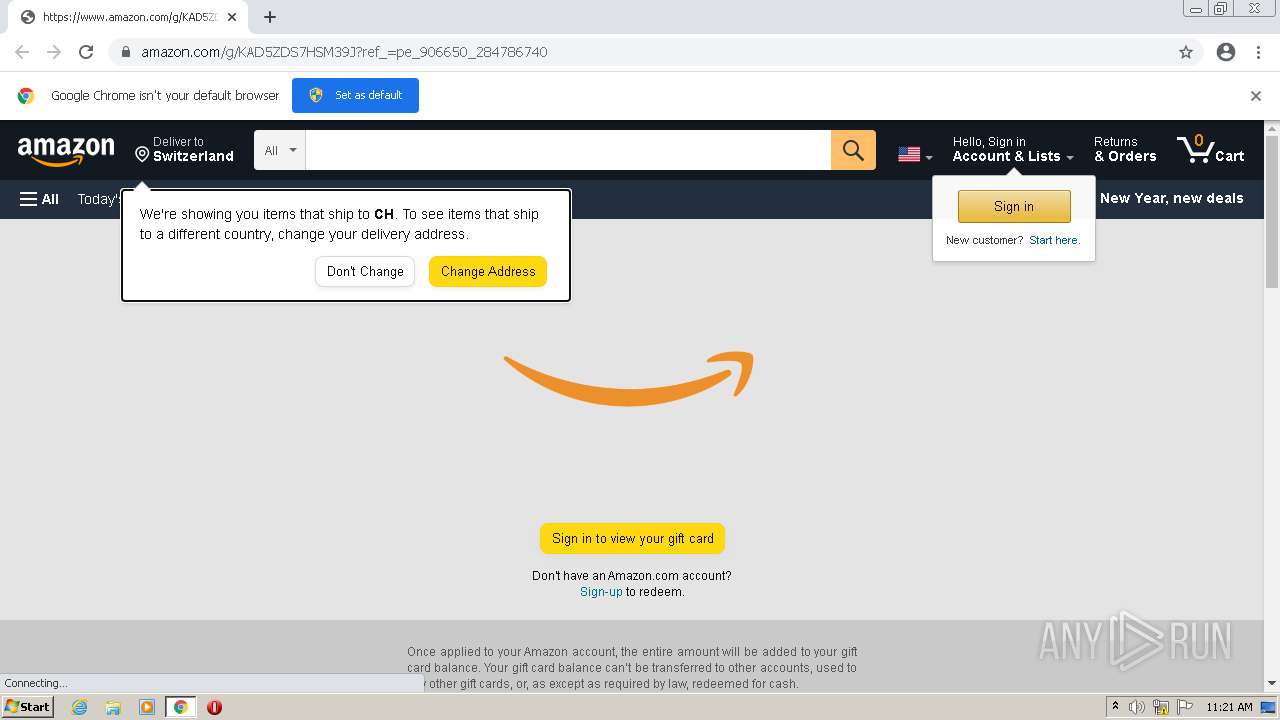This rectangular image is a detailed screenshot of a page on the Amazon website, viewed through the Google Chrome browser. In the top-left corner, a tab displays the URL "https://www.amazon.com" in black text on a white background. Beneath the tab, the Google Chrome icon is visible, along with a message indicating, "Google Chrome isn't your default browser," followed by a blue button labeled "Set as default."

The main content of the screenshot features the Amazon homepage. In the upper-left corner, there is a notification stating, "Deliver to Switzerland." Nearby, there are options to "Hello, sign in," view "Accounts & Lists," and check "Returns & Orders." The shopping cart icon, showing zero items, is also visible.

Central to the image is a white rectangular notification box with black text that reads: "We're showing you items that ship to CH. To see items that ship to a different country, change your delivery address." Directly below this message are two options: "Don't change" in a white box and "Change address" in a yellow box.

The screenshot captures the essence of the user's browsing experience on Amazon, highlighting important navigation and location-based shopping options.